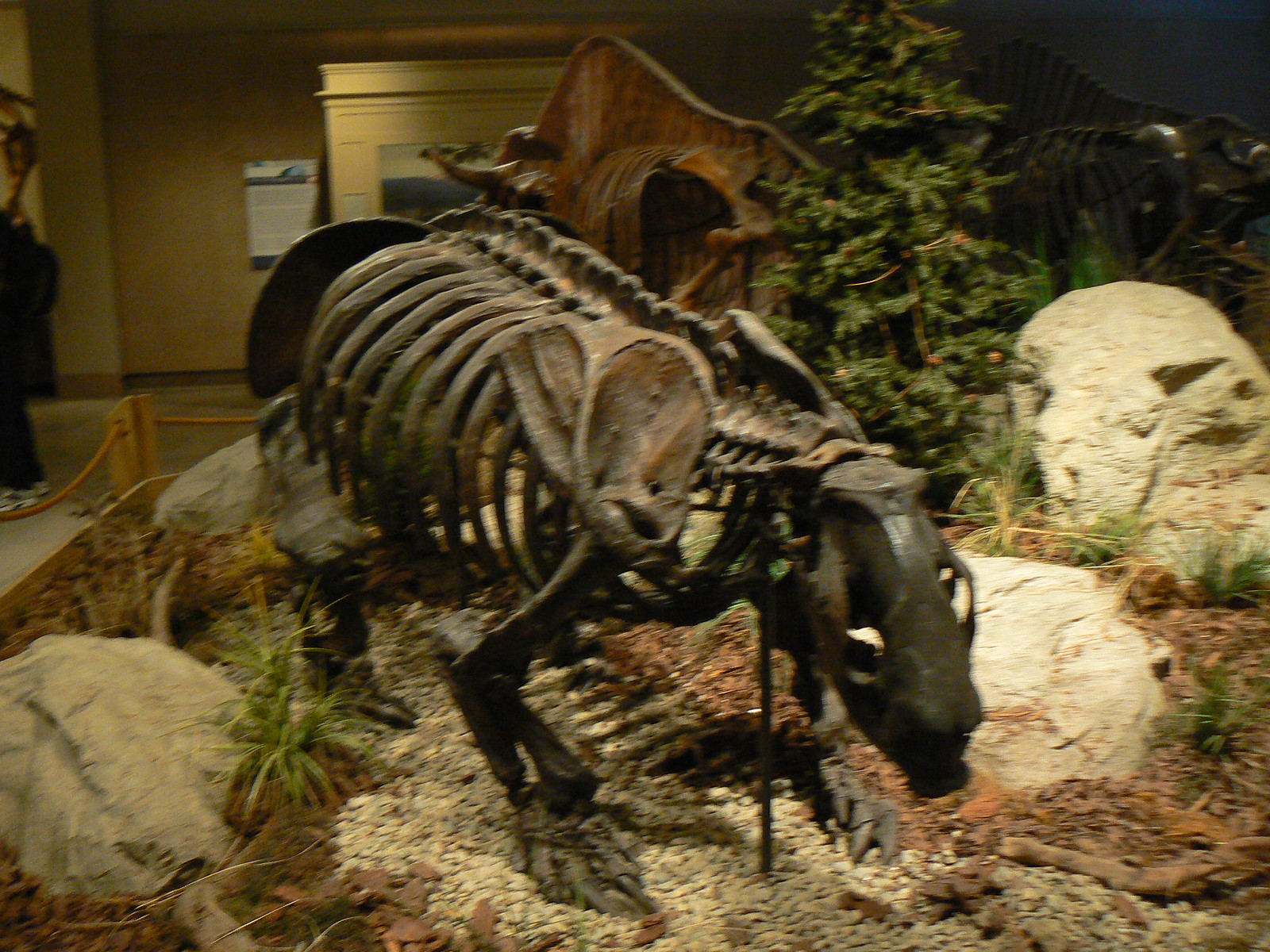The image depicts a detailed indoor color photograph of a Natural History Museum exhibit. The scene is dominated by the dark, fossilized skeleton of a large quadrupedal creature, possibly a bear-like animal, featuring pronounced scapulae and rib bones, with visible claws on its front feet. This imposing skeleton faces the lower right corner of the image. The exhibit attempts to recreate a natural habitat, complete with rocks, boulders, dirt, gravel, and a prominent pine tree at the center. A roped-off area encircles the display, ensuring it remains undisturbed by visitors. The background reveals a brown wall, an archway leading to another section of the museum, and a white sign. Additional darker skeletons of other prehistoric animals are partially visible in the backdrop, with one seemingly exhibiting horns and a taller stature. Sneaker-clad feet of a person are also faintly visible toward the back of the display.